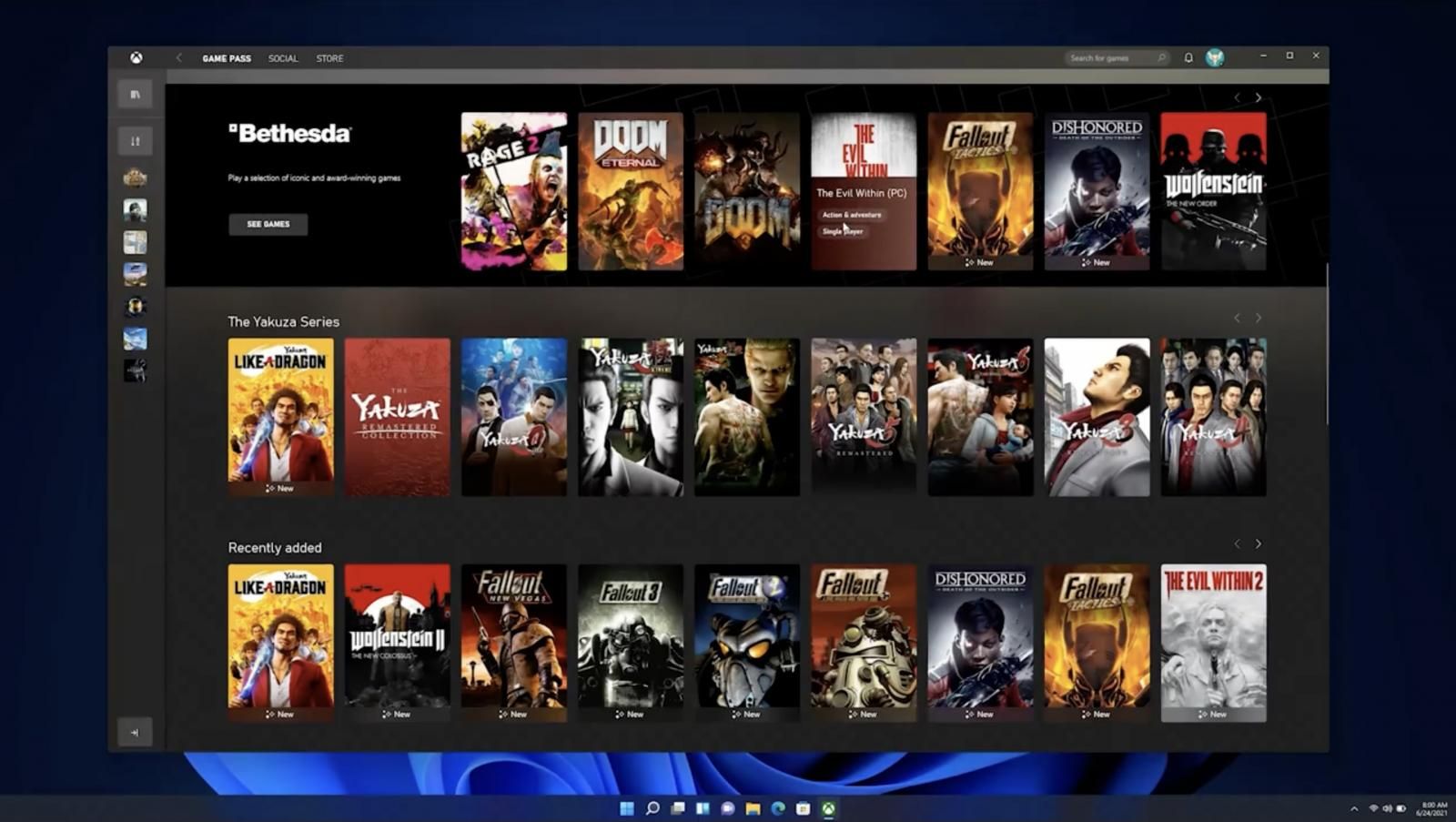The home screen of a game streaming service, resembling Xbox Game Pass, is displayed. The interface features three horizontal rows of game thumbnails, each displaying nine titles. The top row is branded "Bethesda" and showcases games such as Rage 2, Doom, Doom 3, The Evil Within, Fallout, Dishonored, and Wolfenstein. The second row highlights the Yakuza series, including titles like Yakuza: Like a Dragon and several other entries in the Yakuza franchise. The third row is labeled "Recently Added."

At the top of the screen, there are menu options including Game Pass, Social, Store, Search for Games, along with standard alerts and options for saving and exiting. Along the left-hand side, a vertical column likely displays icons for different user profiles. A blue ribbon-like banner stretches across the bottom of the screen, and the overall border of the interface is black.